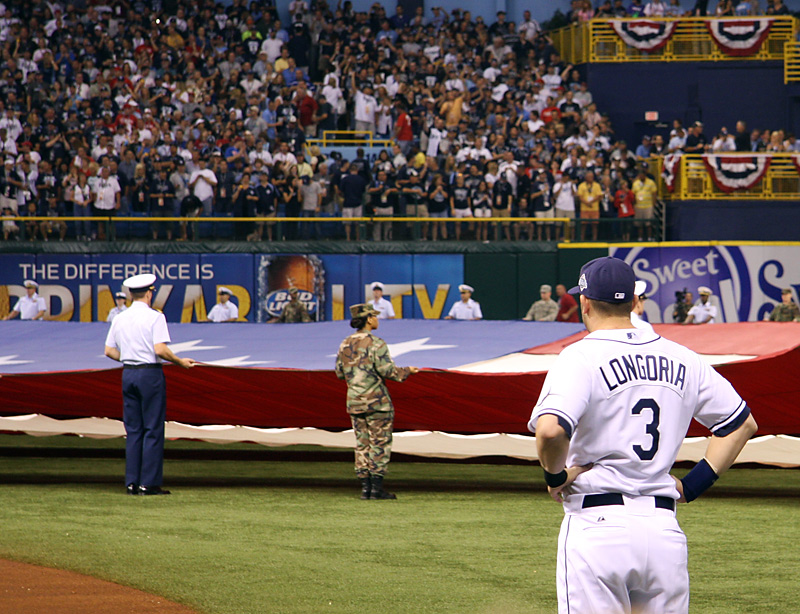At the start of a baseball game, servicemen and women in camouflage uniforms and dress blues, with crisp blue pants, white shirts, and flat-topped Navy hats, hold a large U.S. flag on the field. A banner behind them reads "The Difference is Driven" against a blue backdrop. Above, red, white, and blue banners adorn the yellow balcony seats. Fans in the stands stand with their hands over their hearts, some capturing the moment on their phones. A baseball player, Longoria, prominently stands in the foreground wearing a white uniform with the number three and his name outlined in black on his back, along with a blue baseball cap. A Bud Light sign is also visible, adding to the stadium's vibrant atmosphere.